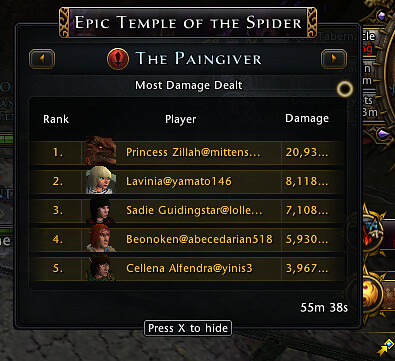The image features a dark, mostly black square with gray highlights and lines, overlaid with a detailed UI reminiscent of a video game, possibly for a PlayStation or PC. At the top, a prominent banner with gold accents on the ends reads "Epic Temple of the Spider" in bold white letters. Directly beneath it, in a serif font, is the title “The Paingiver” accompanied by a red ruby icon. Flanking this title are paging arrows. Below “The Paingiver,” a subtitle reads “Most Damage Dealt.”

The central part of the image is dominated by a detailed table listing player ranks. The table has three columns: Rank, Player, and Damage. The Rank column lists numbers from 1 to 5. The Player column features digital cartoon avatars alongside names, specifically:
1. Princess Zila at Mittens
2. Lavinia at Yamato 146
3. Sadie Guide Star at Lolly
4. Brielle Noken at Ebiserian 518
5. Selena Elphendra at YNIS 3.

The Damage column displays the corresponding damage values: 20,293; 8,118; 7,108; 5,930; and 3,967. 

At the bottom right corner, there is a timestamp reading 55 minutes, 38 seconds, alongside instructions to “Press X to Hide.” The backdrop remains indistinct, maintaining the focus on the informational UI elements.